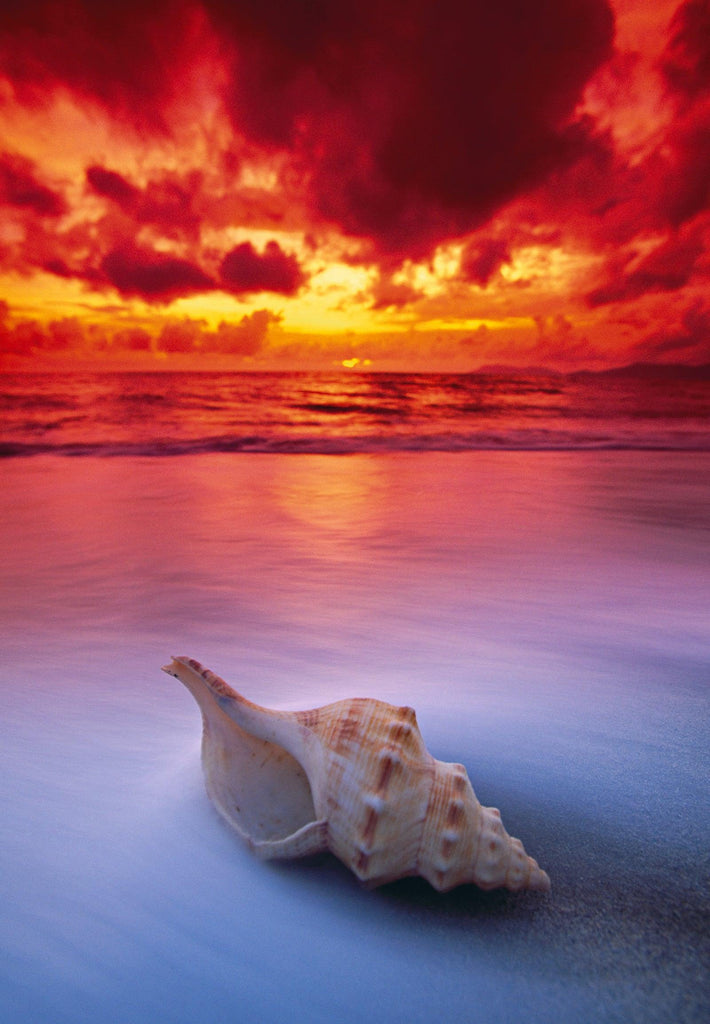This enhanced photograph captures a serene seascape at sunset. Foregrounded by wet, glassy sand tinged in pink and white, the centerpiece is a detailed conch shell with intricate ivory, beige, and brown hues. The shell lies on its side, partially shrouded in a misty blur of water that evokes a foggy haze—a result of the long exposure that gives the water a solid, flowing appearance. Gentle, short waves approach in the distance, their colors deepening into orange and purple as they reach further into the photograph. Above, the sky transitions from a vivid yellow near the slightly elevated sun to a spectrum of dark red and orange clouds, casting a fiery glow over the entire scene. The overall effect is a stunning interplay of natural and digitally enhanced beauty, with rich, harmonious colors that evoke the tranquility and awe of a beach at sunset.